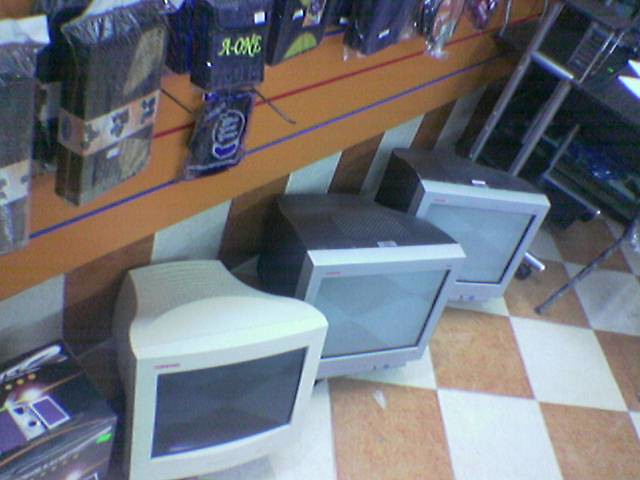In this detailed indoor photograph, the floor is adorned with a distinctive brown and white checkerboard pattern. The walls feature a striking vertical striped design in matching brown and white hues. On the floor, there's a collection of older-style square televisions along with a computer monitor, all positioned in a casual arrangement. The TV on the left is white, while the remaining two are light gray at the front and black at the back. Above these electronics, an orange-colored shelf or table is mounted, holding several objects wrapped in plastic, though their exact nature remains unclear. To the right, there’s a partially visible rack filled with various miscellaneous items. The background wall showcases a vivid design with a red horizontal stripe above a blue one. In the bottom left corner of the image, a smaller square object with a unique design is also visible, adding to the eclectic assortment of items in the room.